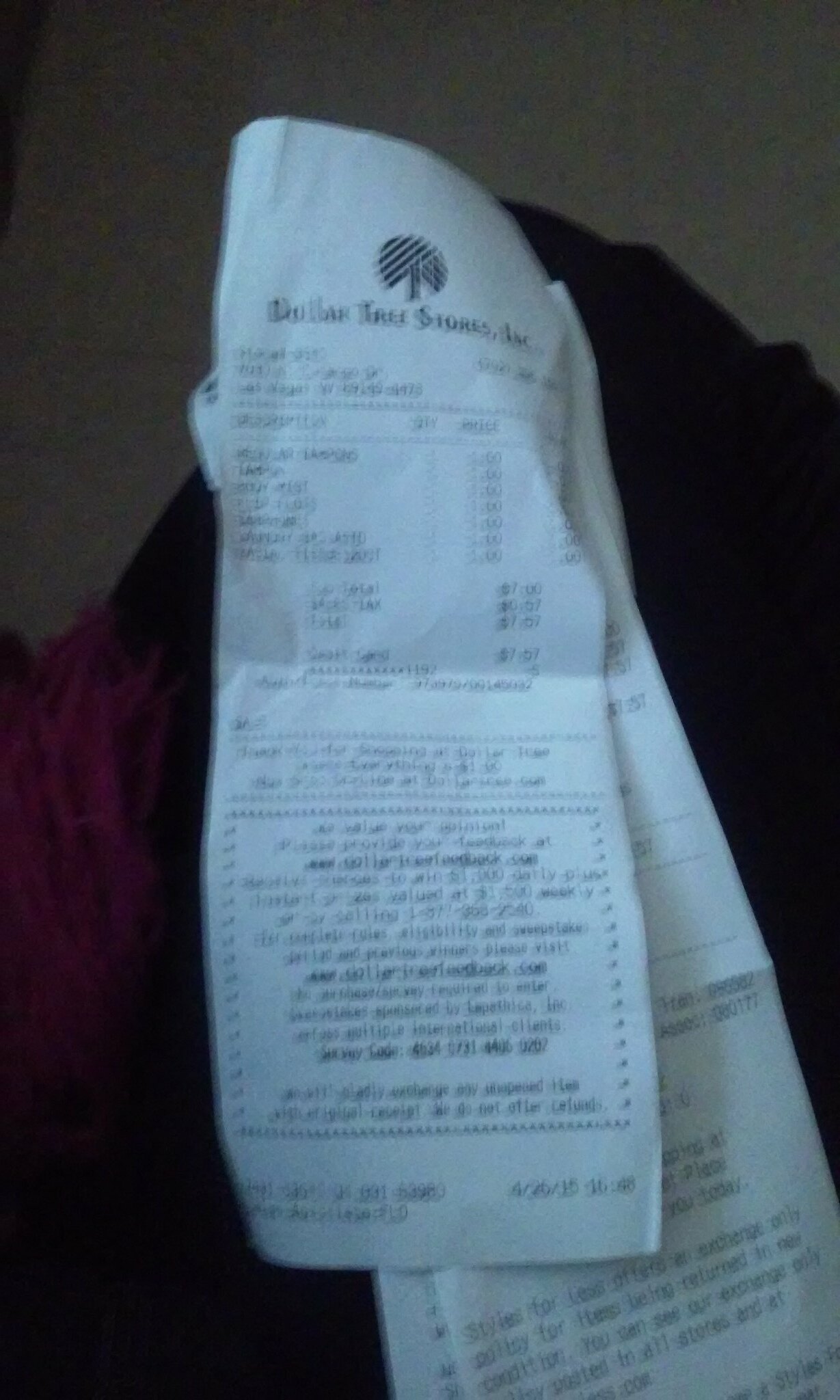A dim and blurry photograph showcases a slightly wadded and wrinkled Dollar Tree Stores Incorporated receipt printed on thermal paper. The receipt sits atop two other partially visible receipts, adding to the layered texture of the scene. Positioned on a dark, shadowy shape against a darker gray surface, the receipt's details are largely obscured by blur, making it difficult to discern most of the words and numbers on it. However, it is evident that a total of seven items were purchased, summing up to $7.57. The bottom portion of the receipt displays a series of words, though they are illegible due to the blurriness.